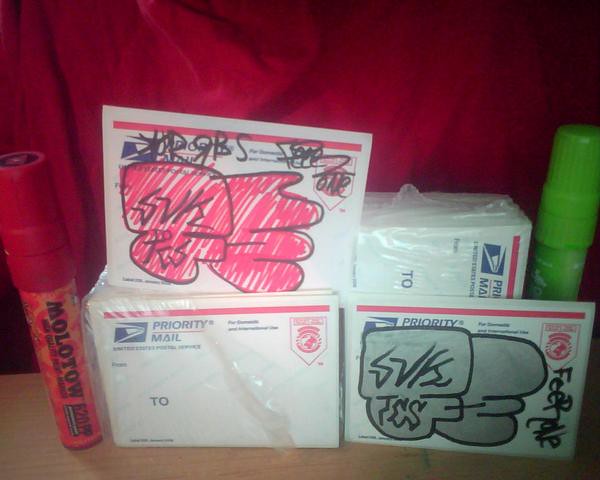This photograph captures a scene featuring several large USPS bubble mailers, each with the USPS logo at the top left and "Priority Mail" in blue text. These mailers are arranged on a light wooden surface, partially framed by a red fabric backdrop that resembles a curtain. Prominent in the scene is a red marker labeled "Molotow" positioned upright on the far left, hinting at its association with street art or graffiti. Among the mailers, two feature colorful, cartoon-like drawings with accompanying text. One of these displays a red hand-like image, while another appears to have a gray hand motif. Behind these illustrated mailers, there is a lime green marker or spray can. The composition suggests a mix of mailed parcels and artistic tools, blending functionality with creative expression.